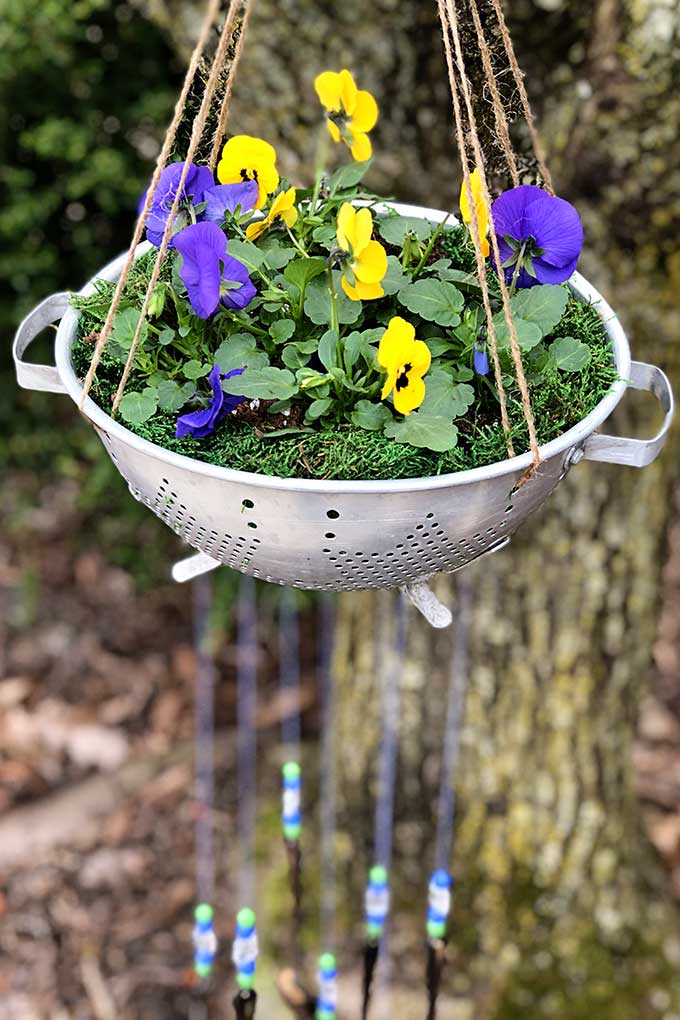This compelling color photo was taken outside, possibly in a home garden, featuring a creative DIY hanging planter. The focus of the image is a repurposed silver colander, utilized as a planter which is artfully suspended by four strands of brown twine from a mossy tree branch that splits into two forks. Inside the colander, there are vibrant pansies, predominantly with a mix of around six yellow blossoms centrally located and approximately four purple ones, along with an additional purple pansy on the right side. The soil and moss medium within the colander helps retain moisture for the flowers. The rustic scene is enhanced by strands of beads in green, blue, and white hanging from the pot, adding a decorative touch. The background is blurred, showing hints of garden elements like grass or vines, dirt, and possibly another shiny object. This charming image showcases both the beauty of nature and the ingenuity of eco-friendly gardening.